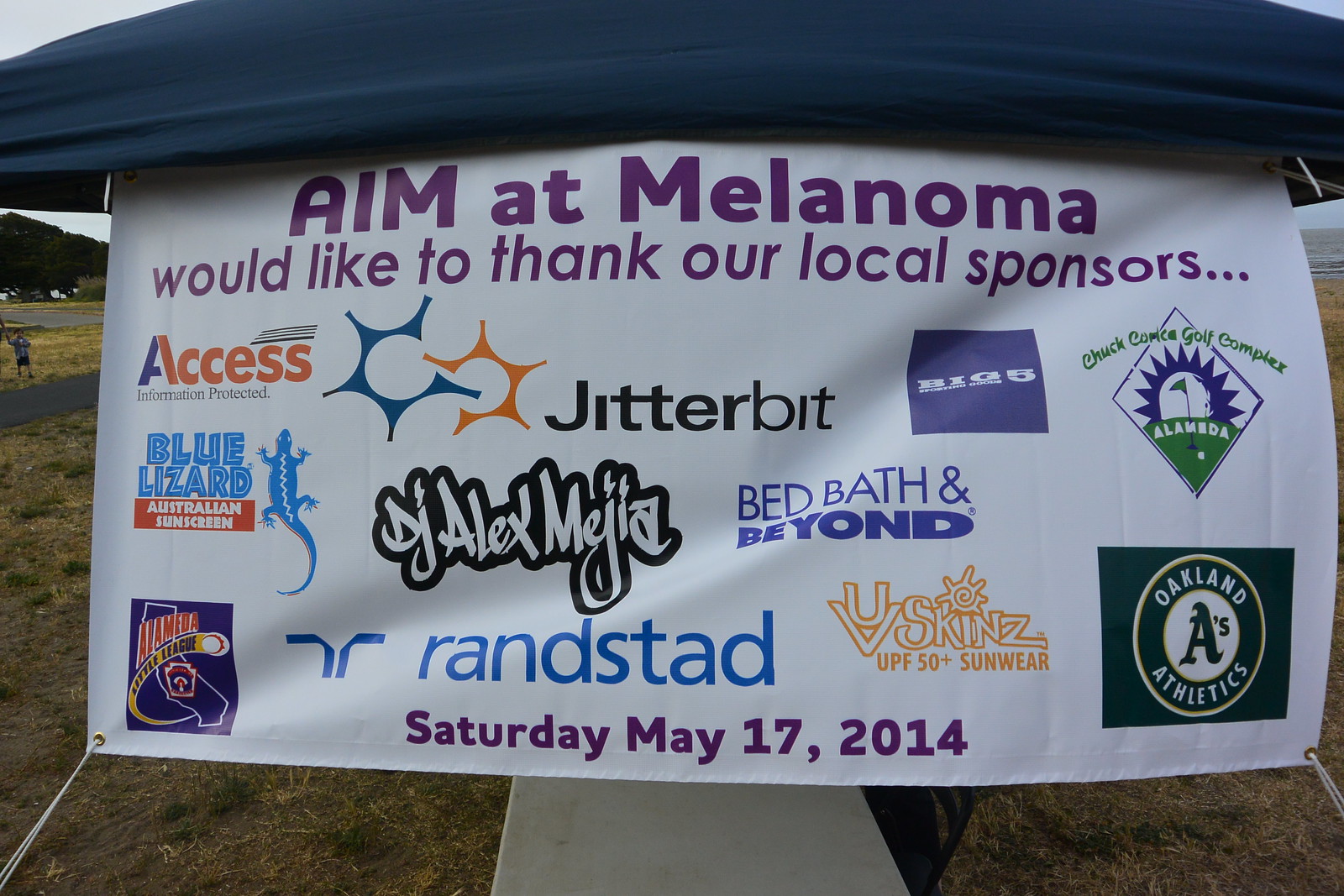This image features a horizontally-oriented white banner tied to a blue tent, situated in an outdoor setting, with visible green grass and a background indicating a park or field. At the very top in bold purple letters, it reads "AIM at Melanoma." Beneath this, it states, "Would like to thank our local sponsors..." followed by several corporate logos and names. Notable sponsors include Access, Blue Lizard (with an icon of a blue lizard and the text 'Australian Sunscreen'), DJ Alex Meja, Randstad, Jitterbit (accompanied by two five-pointed stars, one blue and one orange), Bed Bath & Beyond, Big Five (displayed within a blue square), Chuck Comic Golf Complex, Oakland Athletics, and UV Skins UPF 50+ Sunwear. At the very bottom of the banner, in purple letters, it notes, "Saturday, May 17, 2014." The banner is prominently displayed, tied securely with a white string, and photographed facing the camera.